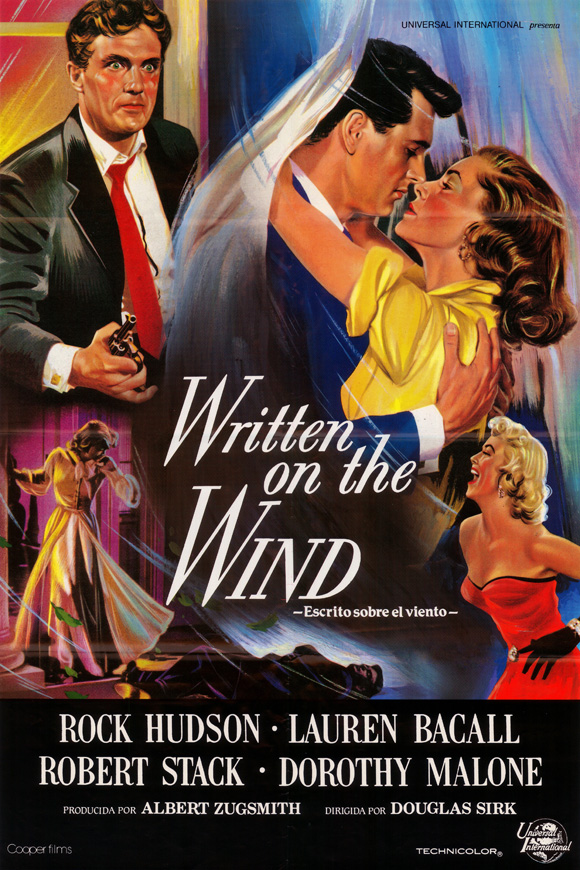This detailed, vintage movie poster for "Written on the Wind" features vibrant, full-color illustrations of the film's characters. At the top left, a man in a black suit with a red tie and brown hair is prominently pictured, poised with a pistol aimed forward. To the right, a couple shares a tender moment, with the man in a blue suit and black hair just about to kiss the woman in a yellow dress and brown hair. Below, the scene transitions to a woman with white blonde hair in a striking red dress, her shoulders bare and a playful smile on her face. Another woman in a long white gown with long brown hair stands elegantly to the left. Centered in white text is the film's title, "Written on the Wind," followed by a black band displaying the names of the stars: Rock Hudson, Lauren Bacall, Robert Stack, and Dorothy Malone. Detailed credits at the bottom include mentions of Albert Zucksmith as producer, Douglas Sirk as director, and Universal International's Technicolor branding and emblem. The Spanish translation of the title, "Escrito Sobre el Viento," and distribution mentions of Cooper Films complete the intricate design.